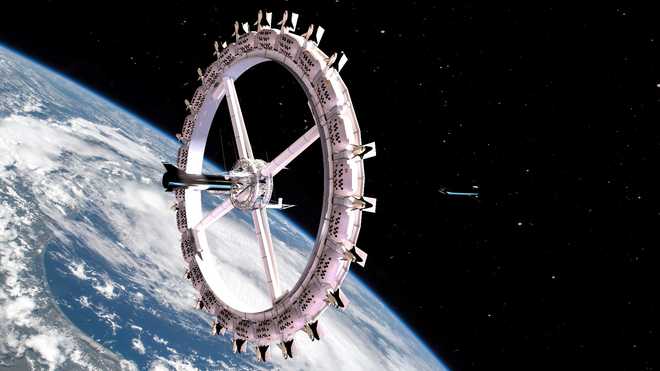This captivating horizontal-rectangular image is set in the vast expanse of outer space. Dominating the lower left portion of the picture is the Earth, partially visible with its vibrant blue oceans, light brown land masses, and wispy white clouds circling its atmosphere. The rich details of the planet stand out against the stark, black void of space that envelops the rest of the scene. 

Central to the image, slightly off towards the middle left, is the International Space Station (ISS). The ISS presents itself as a large circular structure resembling a giant white wheel with a hub at its center, connected by four spokes forming a cross. Along the periphery of the wheel, small projections are spaced intermittently, illustrating the station’s intricate design. Some projections, however, are not visible, as the wheel is partly obscured.

In addition to the ISS, there is another intriguing object—a flat, UFO-like ship—hovering in space, contributing to the futuristic ambiance. Both spacecraft appear to be floating effortlessly, orbiting above the majestic curvature of the Earth. The black sky provides a stunning backdrop adorned with tiny, distant stars, emphasizing the enormity and mystery of the cosmos.